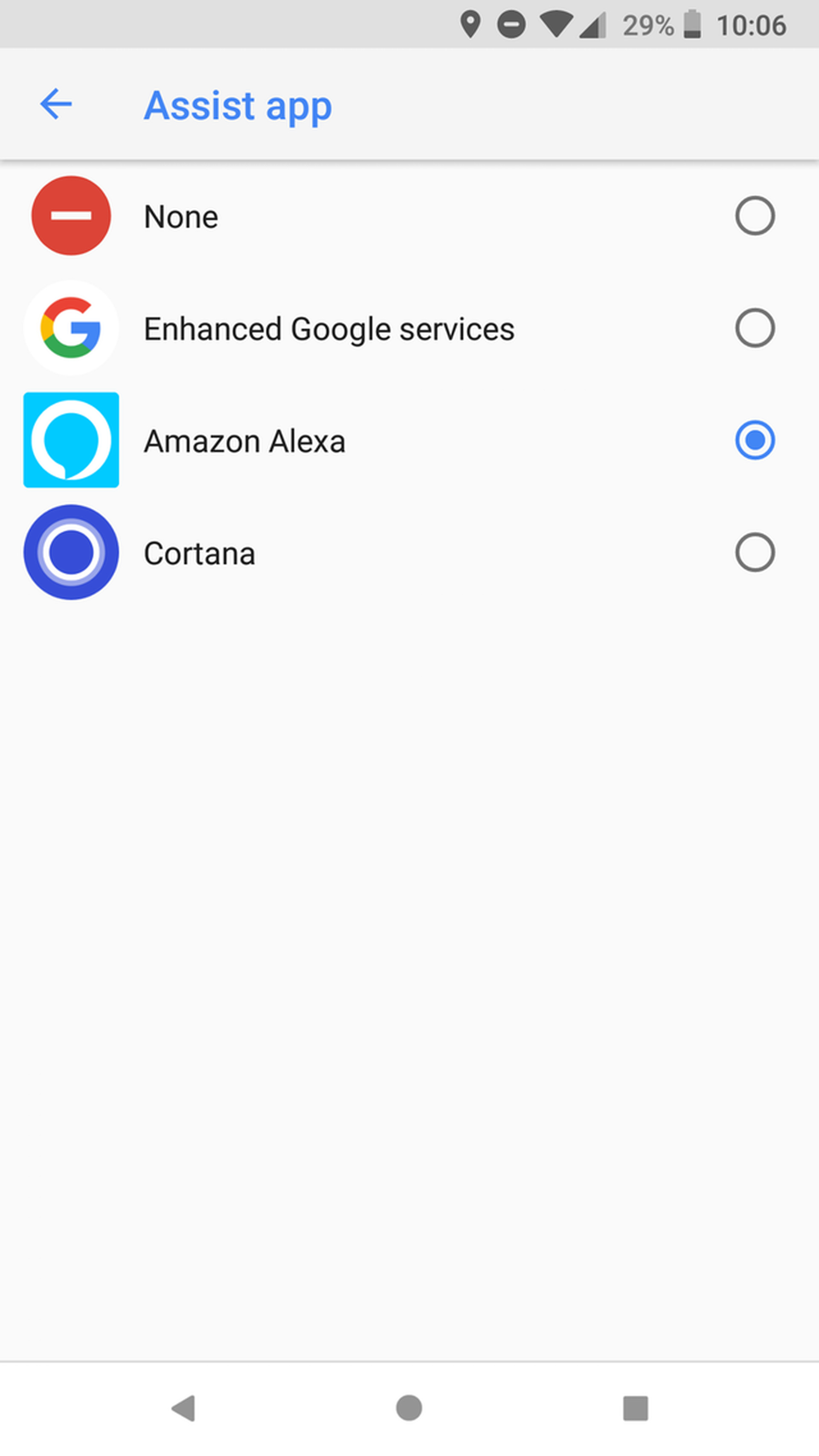A screenshot from a cell phone is displayed, featuring various interface elements. The top of the screen is dominated by a light gray notification bar. The status icons from left to right include: location services enabled, 'Do Not Disturb' mode active (indicated by a circle with a white minus sign in the center), a fully populated Wi-Fi signal icon, and a cellular data signal showing two-thirds strength. On the right side of the notification bar, the time is shown as 10:06, with an adjacent battery icon indicating a nearly drained battery, with just a small amount of charge remaining at the bottom.

Beneath this notification bar, there's a section highlighting assistant applications. The left side features a labeled section "Assistant App," which is followed by a red circle with a minus sign (indicating 'None'), the Google logo for enhanced Google services, the Amazon Alexa logo, and the Cortana logo. The Amazon Alexa icon is highlighted, signifying it is the selected assistant. Below this, an arrow pointing to the left accompanies the text "Assist App," which is displayed in blue, reiterating the selected status of Amazon Alexa.